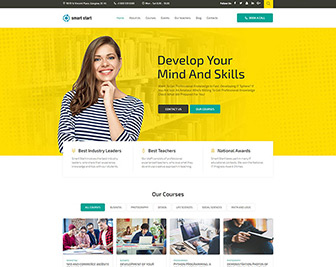A detailed and cleaned-up caption for the described image:

"A web page with a sleek black banner at the top featuring the company's name (unreadable) in black text. The banner includes social media sharing options like Facebook and Twitter, alongside other text too small to discern. Below the banner, the company name is displayed in black on a white background, accompanied by a blue icon. There are several gray text options to the right, also too small to read, and a green action button, possibly to contact the company. 

The main content section has a mustard yellow background showcasing an image of a smiling woman with long, light brown hair. She's dressed in a blue and white, horizontally striped long-sleeve shirt with a boat neck. To her right, the text 'Develop Your Mind and Skills' is prominently displayed in black. Beneath this, additional black text and two buttons (one black, one blue) are present, but the text is too small to read. Further content with similarly small text is situated underneath this section."